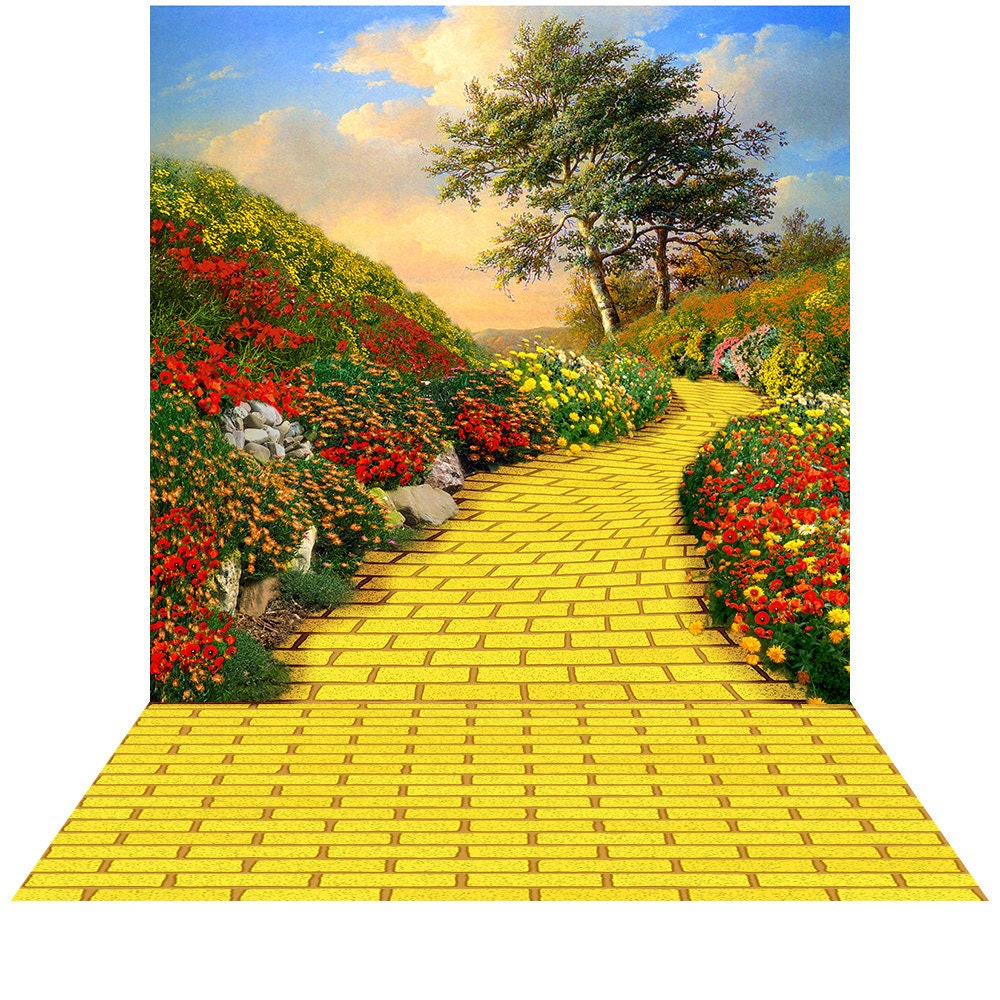This is a vertical, 3D color illustration that creates a striking visual effect, reminiscent of the yellow brick road from "The Wizard of Oz." The image features a yellow brick road that begins as a foreground floor mat with bright yellow bricks and beige mortar, giving it a seamless extension into the illustrated backdrop on the wall. The road curves to the right and then to the left before disappearing behind a flower-covered hillside, enhancing the 3D effect. Vibrant multicolored flowers in shades of orange, red, and yellow border the path, with floral displays continuing up a hill on either side. In the background, the sky is a mix of blue and white puffy clouds, suggesting a setting or rising sun. Two large green trees stand on the top right, adding depth and a touch of nature to the scene. The highly detailed and hand-painted style of the illustration adds to its enchanting, immersive quality.